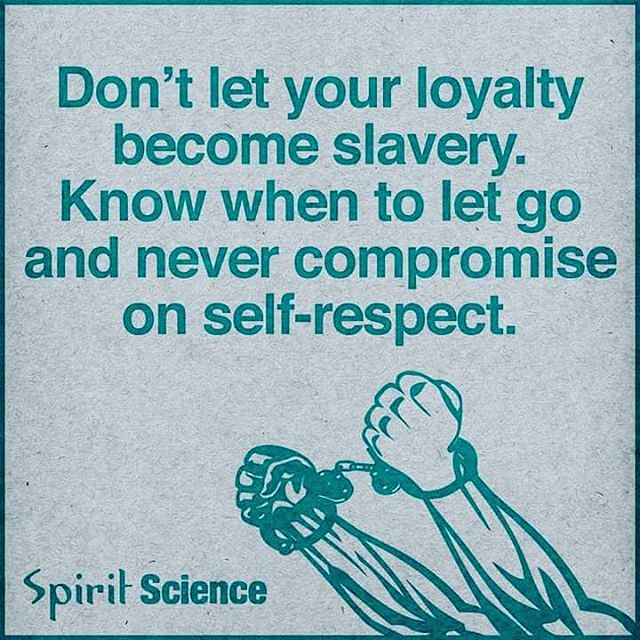The image features a thought-provoking drawing with a poignant message. Set against an off-white, grey background speckled with light green dots, the centerpiece of the artwork is a pair of clenched fists in handcuffs drawn in thick green ink, rising from the bottom right corner. The hands, colored identically to the background, emphasize the tight cuffs around their wrists. At the top of the image, bold green text delivers an inspirational quote: "Don't let your loyalty become slavery. Know when to let go and never compromise on self-respect." The quote is accentuated by the same green color that borders the entire picture. In the bottom left corner, the artwork is signed off with "Spirit Science," grounding the image in its thought-provoking context.